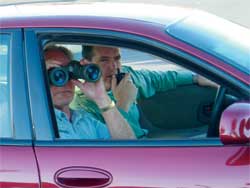The image captures an intriguing scene from the perspective of being level with a four-door, red car viewed through the front passenger side window. The setting appears deliberately staged, suggesting a scene from a TV show, movie, advertisement, or stock photo. The photo is tightly framed, revealing the front passenger window, a sliver of the front windshield, and a glimpse of the back window. The car’s details include a black-trimmed window, a red door handle, and a rearview mirror almost at the edge of the frame. The background is a thin, gray line at the top, with light reflecting off the front windshield.

Inside the vehicle, the window is rolled down, and two men catch the viewer's attention. The man in the passenger seat, closest to the camera, wears a blue button-up shirt, a gold wristwatch, and is intensely peering through a large pair of binoculars. Beside him, the driver, sporting short dark hair and a short-sleeved shirt, has his left elbow resting on the window sill. His right hand is at his mouth, holding what appears to be a walkie-talkie, and his other hand grips the black steering wheel. Their focused gazes suggest they are observing something of importance off to the right, possibly hinting at them being undercover cops.